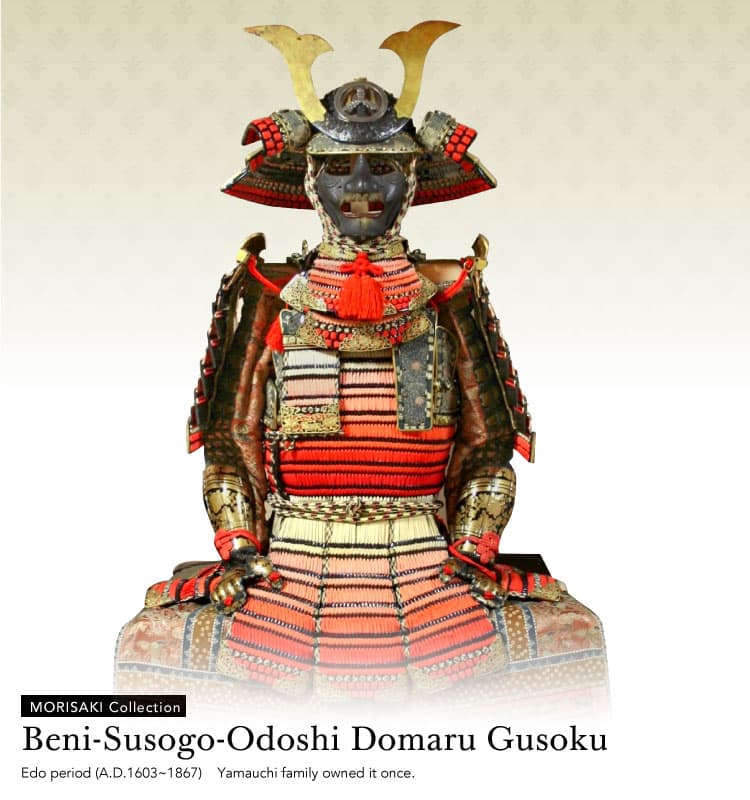The image depicts a detailed statue or a piece of samurai armor, characterized by a grey, metallic faceplate and an ornate headpiece with gold horns. The statue appears to be seated, facing forward with its hands on its legs, dressed in striking, layered clothing that transitions in color from light to orange to red. The background of the image is a smooth gradient from beige to white with a dotted pattern. At the bottom of the image, there is a section of faded text over a rectangular cloth background, with small white text reading "Morisaki Collection." Below that, in black text, the inscription reads "Beni-Susogo-Odoshi-Domaru-Gusoku," indicating that the piece is from the Edo period (AD 1603 to 1867) of Japan and was once owned by the Yamauchi family.